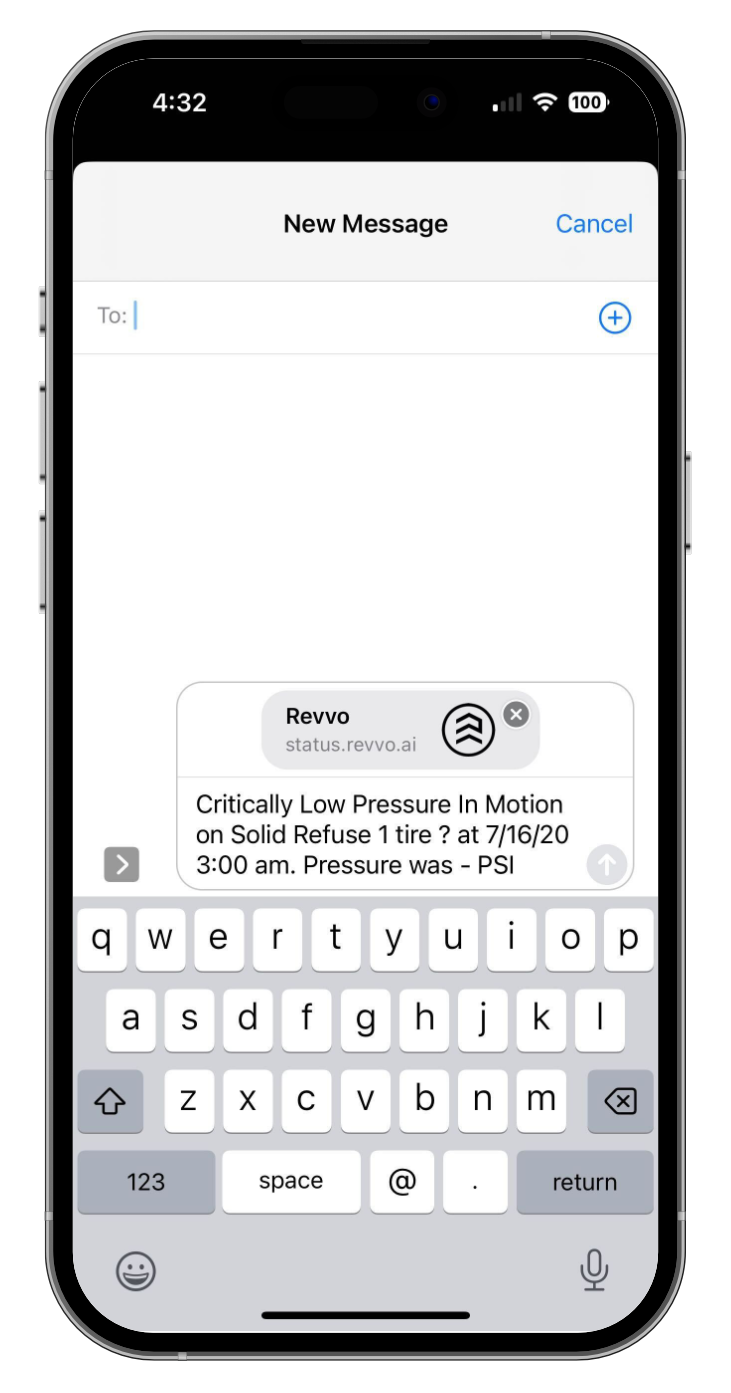The image depicts a close-up of an iPhone screen displaying the messaging app. The device shows the time as 4:32, though it is unclear whether it is AM or PM. In the status bar, the phone has a low cellular signal with only one bar, but it is connected to Wi-Fi and the battery is fully charged at 100%. 

Within the messaging app, a new message is being composed but has not yet been addressed, as the "To" section remains empty. In the message composition area, a link to "revo-status.revo.ai" is being typed, accompanied by the text: "Critically low pressure in motion on solid refuse one tire? 7-16-23 AM. Pressure was minus PSI."

The on-screen keyboard is visible, featuring a smiley face icon in the bottom left for accessing emojis and a microphone button in the bottom right for recording voice messages. The overall design of the iPhone is sleek and premium in appearance.